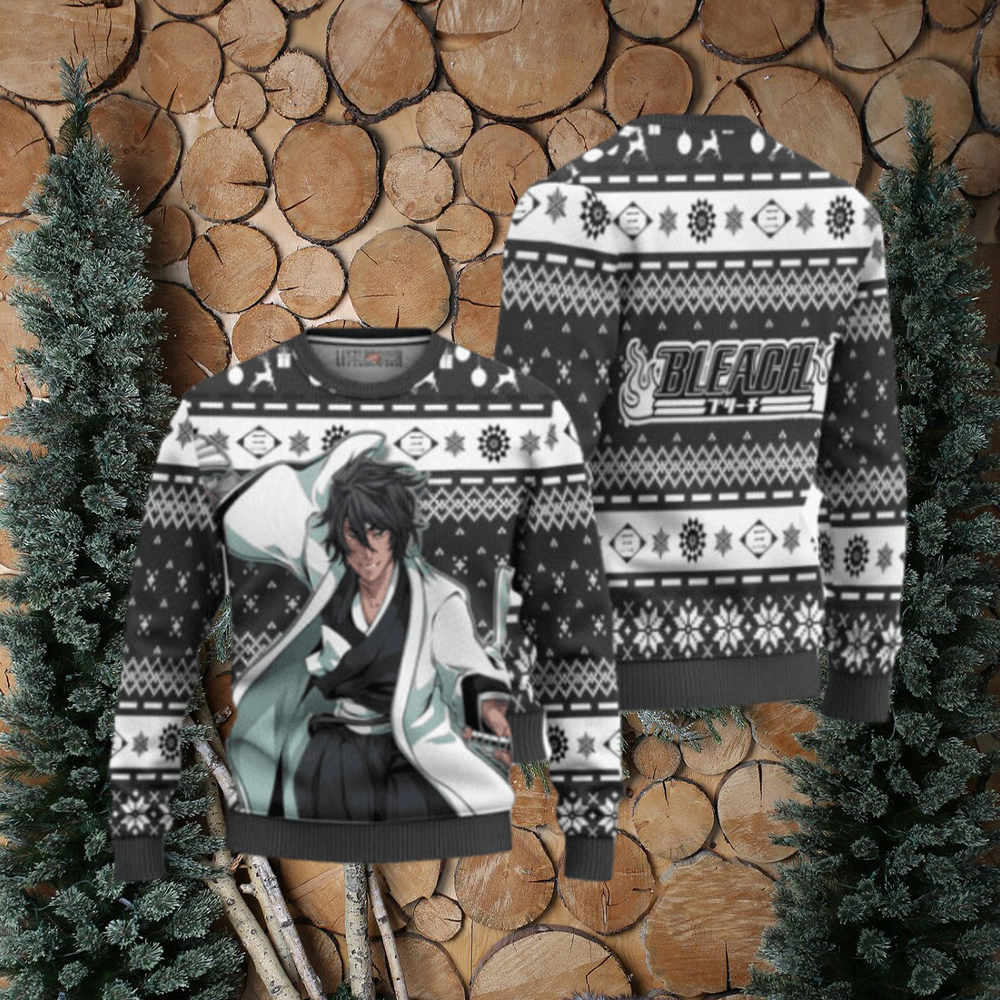In the image, we see a juxtaposition of two gray and white sweaters displayed against a unique background that resembles a collage of stacked firewood discs, punctuated by two artificial pine trees on either side. The sweaters, which seem somewhat blurry and possibly photoshopped, present a front and back view respectively. The front of the left sweater showcases an anime character with black hair, donned in a white robe over black garments, seemingly bursting out of the fabric. This same character is repeated on the back of the right sweater, which also prominently features the word "BLEACH" in all caps black letters, and a number "74". The designs on these sweaters include standard Christmas motifs such as dancing reindeer, black starbursts, and dotted lines, contributing to a conventional yet festive pattern. Additional details like tree branches or walking sticks leaning against one of the artificial trees add a rustic touch to the cozy wintery scene.